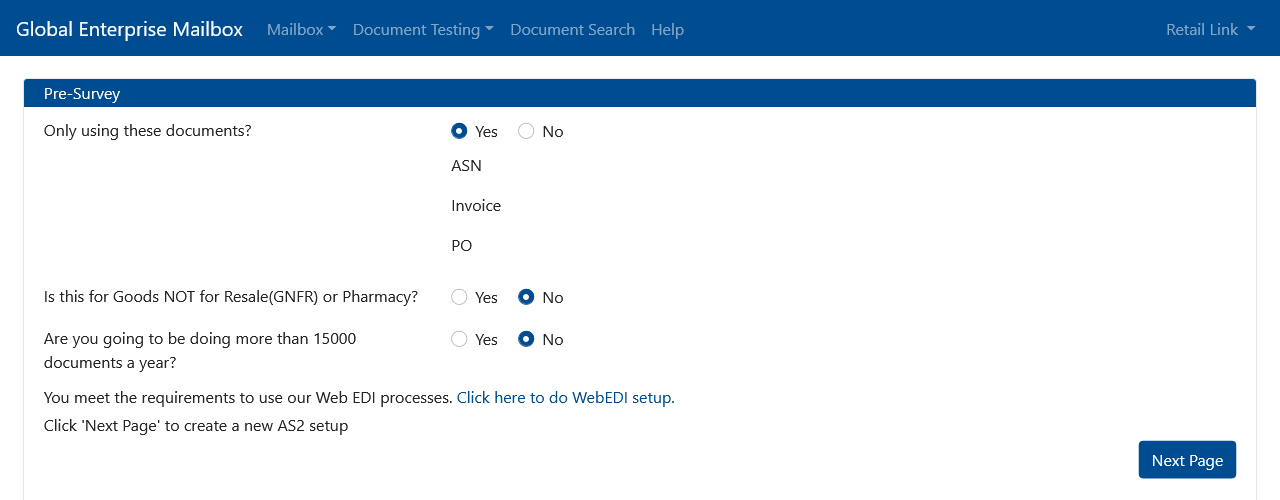This is a detailed screenshot of the Global Enterprise Mailbox desktop application interface, featuring a predominantly blue header with the application name "Global Enterprise Mailbox" in white font at the top left. Adjacent to this, there are four hyperlinks: "Mailbox" (slightly grayed out with a dropdown), "Document Testing" (also with a dropdown), "Document Search," and "Help." To the far right, there is a dropdown menu labeled "Retail Link."

Below the header section, there is a smaller rectangular enclosure also topped with a blue background. This section is labeled "Pre-Survey." The main content area beneath this has a predominantly white background. It features the instruction "Only Using These Documents," accompanied to the right by Yes and No radio buttons, with Yes selected.

Further down, the labels "ASN, Invoice, PO" are listed, followed by a question inquiring, "Is this for goods not for resale (GNFR) or Pharmacy?" Yes and No radio buttons are provided here, with No selected.

Another question asks, "Are you going to be doing more than 15,000 documents a year?" with the Yes and No radio buttons again present and No selected for this question.

Below this, there is a statement confirming, "You meet the requirements to use our Web EDI processes," with a hyperlink to the right instructing users to "click here to do Web EDI setup."

Finally, the interface prompts users to "click Next Page to create a new AS2 setup," with a prominent blue rectangular button labeled "Next Page" to the right.